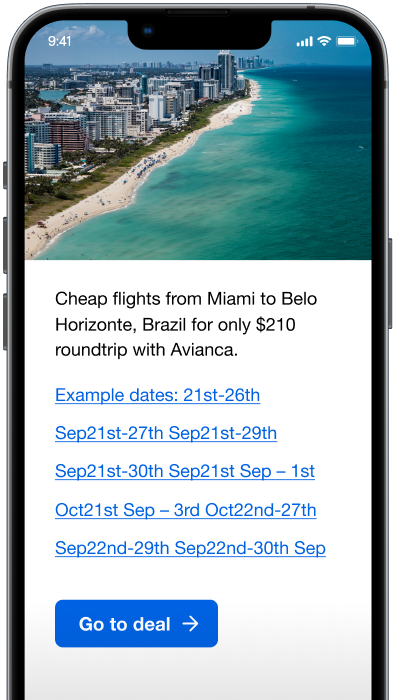The image portrays a close-up of a cell phone screen displaying various details. The phone, appearing considerably large in the frame, shows the time as 9:41 with a fully charged battery and strong Wi-Fi signal. The background image on the phone features a serene ocean scene, including a shore lined with several people, lush grass, and bushes. Beyond the shore, a cluster of tall city buildings stands prominently.

Overlaying this background, a bold text advertisement announces: “Cheap flights from Miami to Belo Horizonte, Brazil, for only $210. Round-trip with Ivankia.” The ad also provides several example date ranges for these flights: September 21st through 26th, September 21st through 27th, and September 21st through 29th, all of which are clickable links. Additionally, another clickable link offers dates from September 21st through 30th, and a final link mentions dates from September 21st to October 21st. The ad conveys all pertinent information clearly and concisely for those interested in booking these affordable flights.